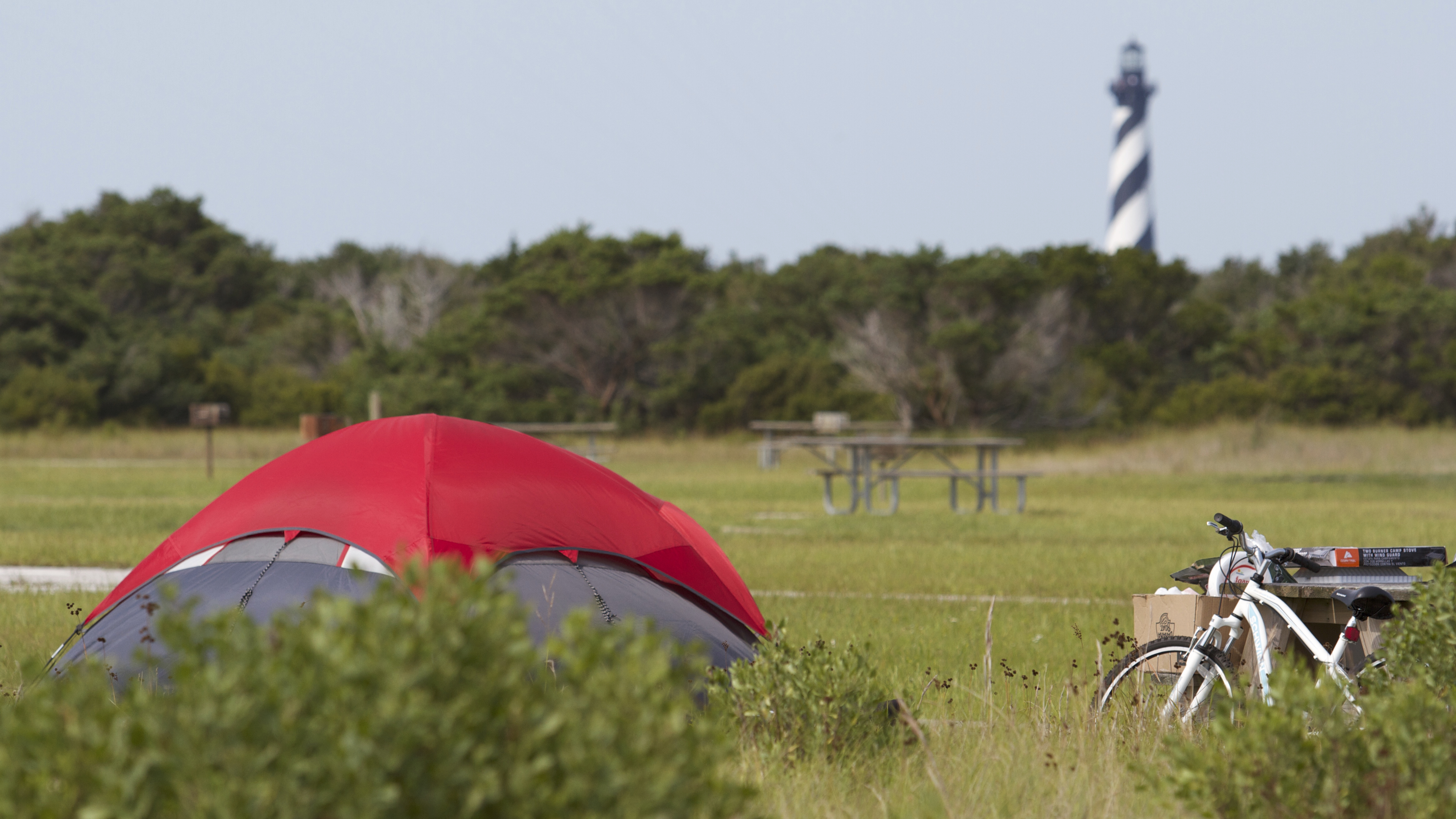This photograph captures a vibrant and picturesque outdoor scene, likely in a public park or campsite. In the foreground on the left side, there is a tent with a striking red rain cover over a gray base, surrounded by dense foliage and some smaller bushes. Adjacent to the tent are various personal items, including potential camping or biking equipment. On the lower right side, a white bicycle is propped against a wooden table or possibly boxes that contain additional items or supplies. Moving further into the image, the middle ground reveals a green, open field that serves as a picnic area, dotted with wooden benches and possibly a barbecue pit. The background is framed by a thick, lush forest forming a dense tree line. A notable feature is a black and white striped lighthouse located about a third of the way from the right side of the image, adding a whimsical touch to the scenery. The sky is clear and blue, indicating a bright day, enhancing the idyllic and peaceful atmosphere of the scene.